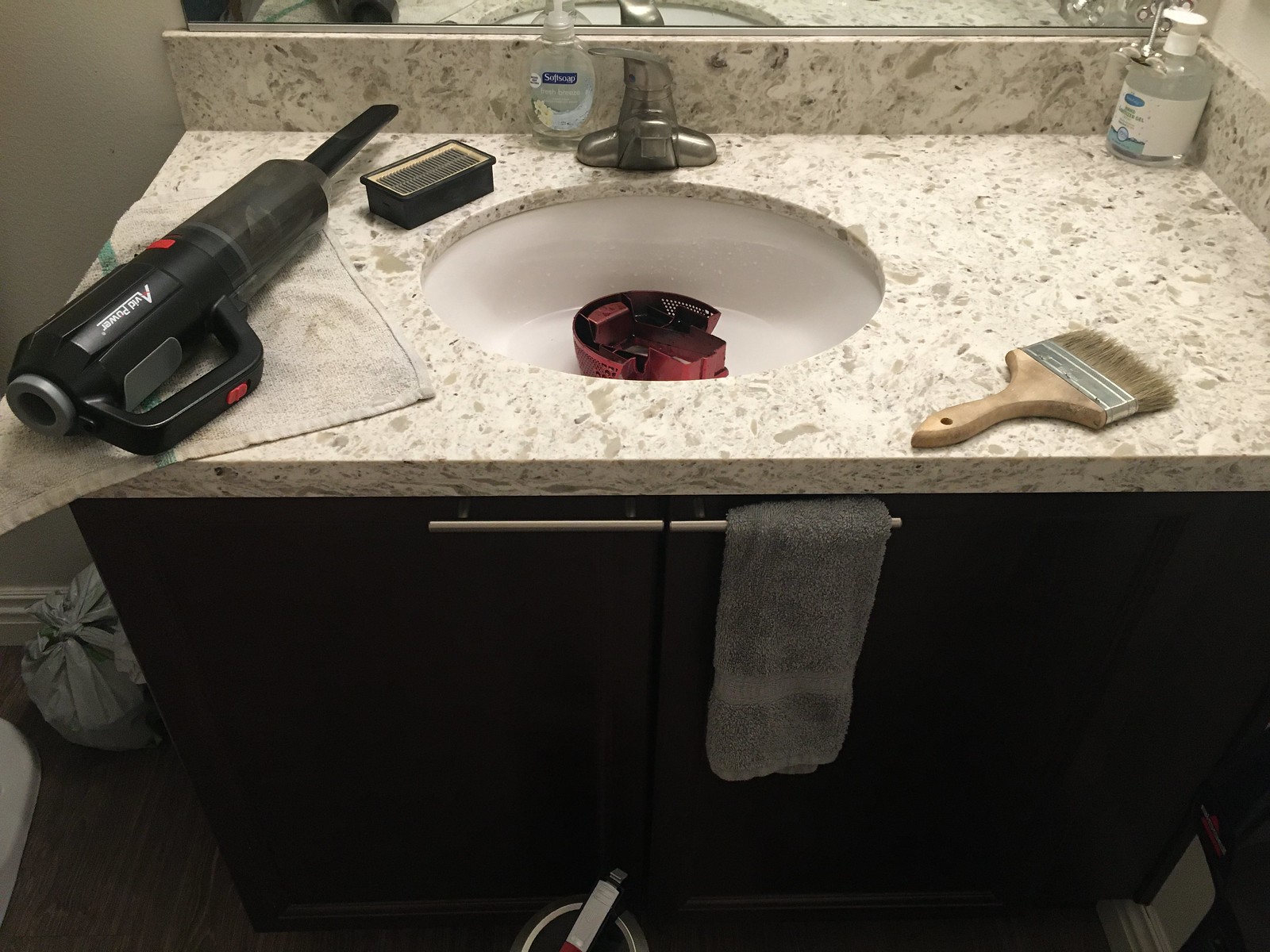The image captures a detailed landscape view of a bathroom sink area. The countertop, made of light tan marble with a richly textured surface, holds several objects. In the far corner of the counter sits a bottle, while to the left of the water faucet, there is a clear plastic soap container adorned with blue writing. The faucet itself is a single-handle, bronzed fixture, exuding an antique charm.

To the left of the faucet, a small ornamental box in black adds a touch of elegance. Within the sink, a mysterious red object lays unidentified. On the counter, to the left of the sink, rests a tan towel with a small, handheld vacuum cleaner placed on top of it.

Further to the right of the sink, near the front, a wood-handled paintbrush is positioned. Its brown handle contrasts with the tan brush bristles, held together by a metal band. The cabinetry below the sink is made of dark wood and features two silver handles directly below the sink; a gray towel hangs neatly from one of these handles.

On the floor, to the left of the cabinet, a tied-up tan plastic bag can be seen, completing the scene with a touch of everyday practicality.